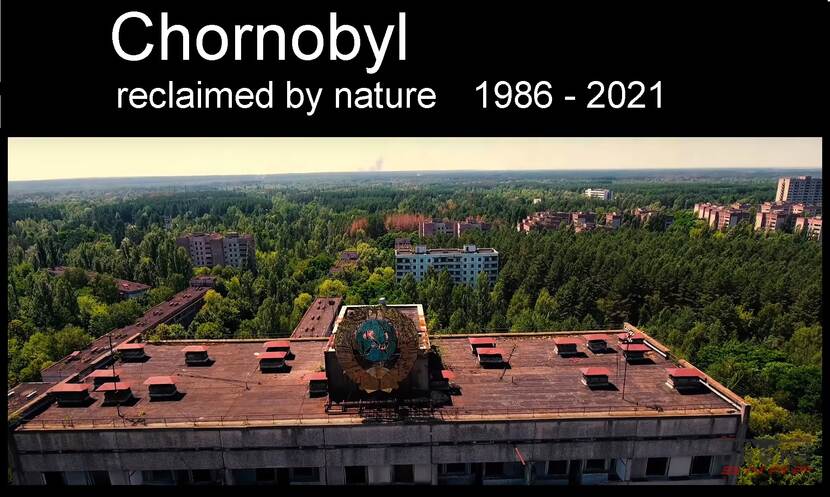This photograph, apparently taken from a drone, captures a striking view of Chernobyl, vividly illustrating its reclamation by nature between 1986 and 2021. At the uppermost section of the image, a label reads "Chernobyl Reclaimed by Nature, 1986-2021," highlighting the transformation of the site following the infamous nuclear disaster. The main part of the image offers an aerial perspective, slightly cropped, predominantly showcasing the roof of a building. This rooftop is speckled with red solar panels and, intriguingly, features what appears to be a faux globe at its center, along with a small box structure likely serving as access to lower floors. Surrounding this building are several light-colored, abandoned, and decrepit structures, all enveloped by a dense forest of verdant trees, epitomizing nature's resilience. To the left, the distant highways with occasional cars hint at remnants of human activity, while the right side is dominated by an expanse of more trees under a sky tinged with a yellow hue, suggesting a serene moment of sunrise or sunset. This powerful image encapsulates the eerie yet beautiful resurgence of nature in a once devastated area.